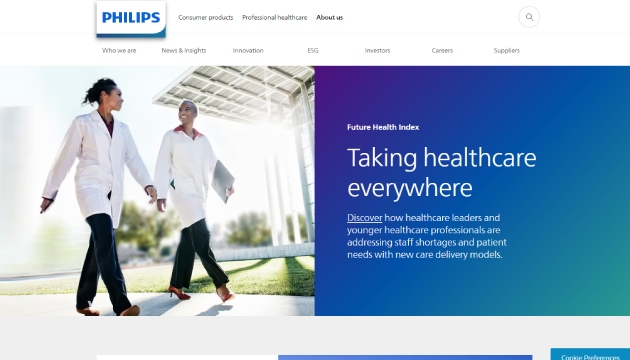This image features a section of a computer screen showcasing the Philips brand interface. The Philips logo, written in blue, is prominently displayed within a white, rectangular box that includes a blue bottom border. Adjacent to the logo, clickable menu items are listed: "Consumer Products," "Professional Health Care," and "About Us." There is also a search icon, represented by a magnifying glass within a circle.

Directly below this menu, additional navigation options are presented in a horizontal layout: "Who We Are," "News and Insights," "Innovation," "ESG," "Investors," "Careers," and "Suppliers."

The main section of the display features an image of two women of color engaged in conversation while walking towards the right side of the screen. Both women are dressed in long white lab coats, black pants, and red shoes. They hold what appear to be folders or laptops down by their sides as their arms swing naturally.

To the right of this image, within a blue box adorned with white text and a faint green gradient in the bottom right corner, is the title "Future Health Index." Below this, the text reads: "Taking health care everywhere. Discover how health care leaders and younger health care professionals are addressing staff shortages and patient needs with new care delivery models."